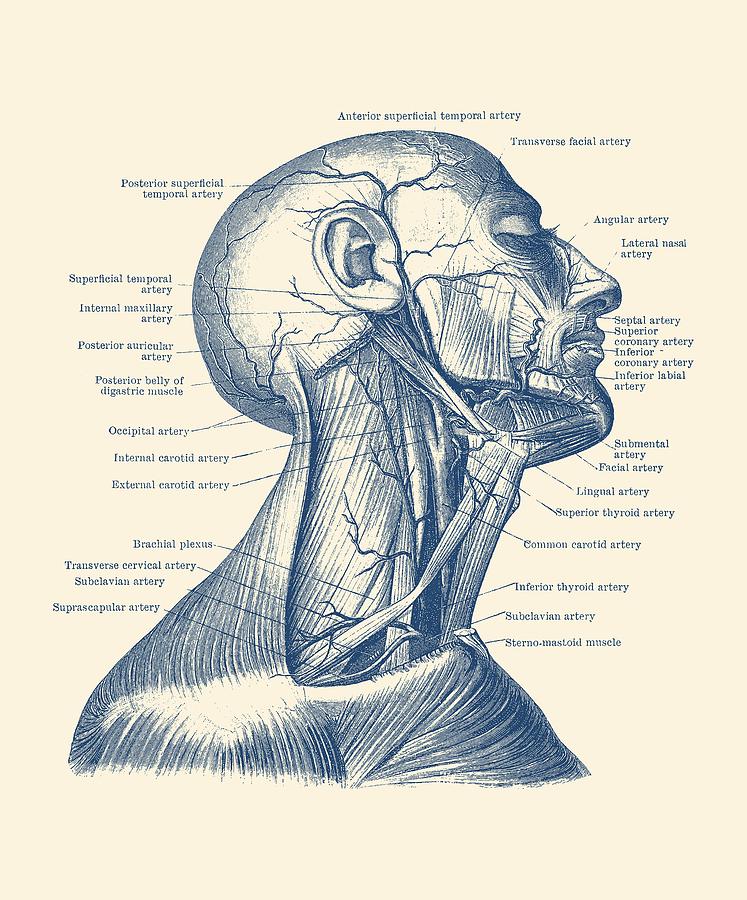This detailed informational poster features a pink background and a black sketch of a bald man's head and neck in profile, with his skull cracked and skin removed to reveal the underlying structures. It showcases the intricate anatomy beneath the skin, including exposed muscles, arteries, veins, and tendons. Both sides of the poster are densely labeled with small bits of text and lines pointing to various anatomical features, identifying critical areas such as the suprascapular artery, transverse cervical artery, brachial plexus, external and internal carotid arteries, occipital artery, sternomastoid muscle, subclavian artery, inferior thyroid artery, and common carotid artery. The man’s neck appears to be laid open, further illustrating the detailed network of blood vessels and muscular systems present in the head and neck region.